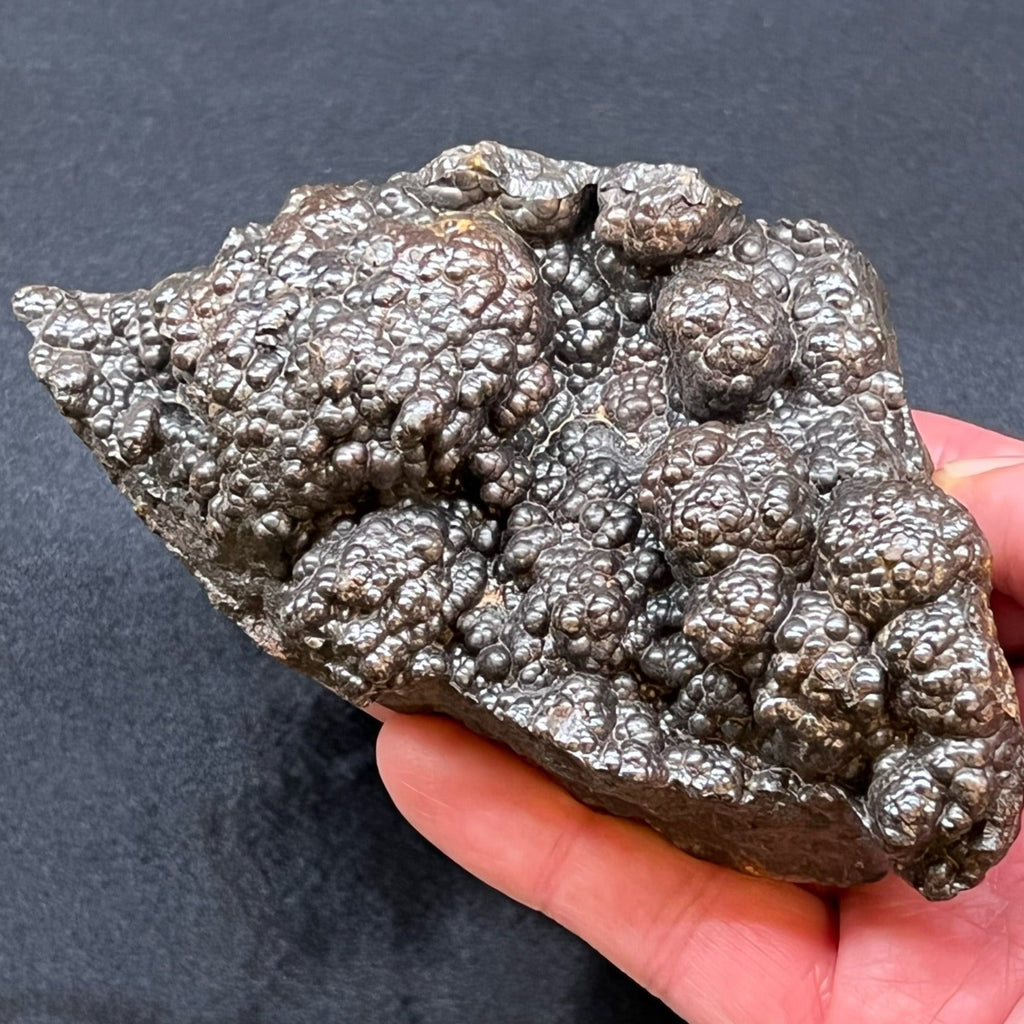In this detailed image, a close-up captures a person's hand, likely Caucasian, holding a fascinating piece of volcanic rock that is semi-reflective under bright lighting. The irregularly shaped rock, approximately the size of the palm, features a striking array of boils, bubbles, and clusters, giving it a textured surface that resembles foam or ash burned and then cooled. The rock showcases an intriguing mix of colors including black, bronze, dark cobalt, and hints of red and gray, enhancing its ancient and weathered appearance. The background is a flat, likely black, slightly shiny surface that could be blue felt, providing contrast and drawing attention to the well-lit bumpy object. The image captures the essence of the rock's geological significance and its captivating bubbled texture.